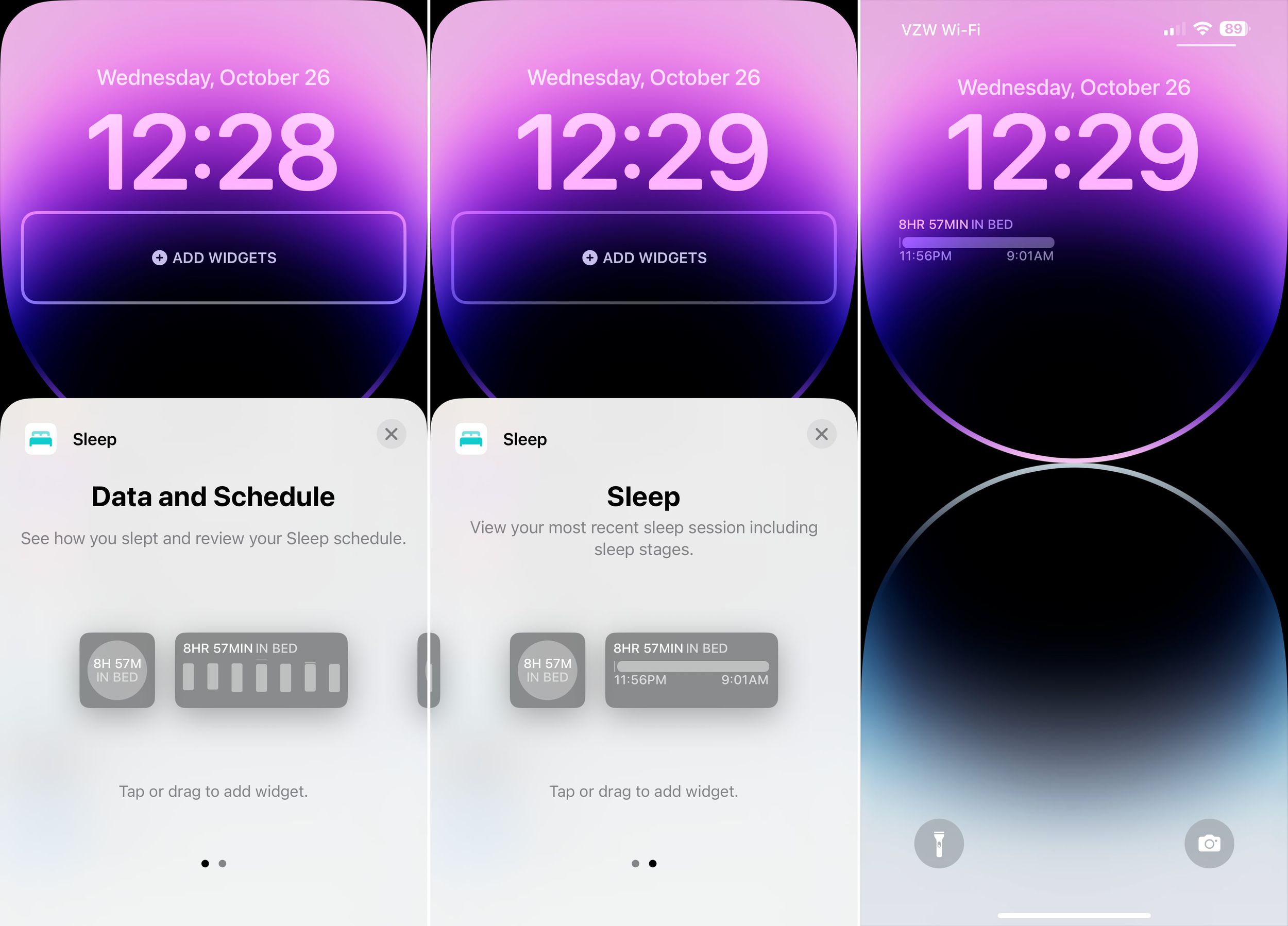The image contains three detailed views of an iPhone, arranged from left to right, each highlighting different aspects and features of the device.

- On the left, the iPhone displays a screen in sleep mode. The date and time are shown as "Wednesday, October 26th, 12:28." The screen predominantly features a sleep widget with the message: "See how you slept and review your sleep schedule," indicating that the user can monitor their sleep patterns.

- The middle view shows the entire front of the phone, which exhibits a captivating gradient design. The colors transition seamlessly from a light lavender at the top to a deeper purple, and then into black towards the bottom. When inactive, the screen showcases two semi-overlapping circles— the top one in purple, and the bottom one in green— set against a backdrop that fades from black to a bluish hue, finally merging into a cloud-like white at the base. The aesthetic is serene and visually appealing, likely designed to evoke a sense of calmness.

- On the right, the iPhone screen reveals a detailed sleep session summary. This view allows the user to delve into their recent sleep session, including the various stages of sleep. The information is presented under the header "Sleep Mode: Just Sleep," with interactive elements that can be tapped and dragged for more detailed insights, enabling users to review their nightly sleep data.

This sequence effectively showcases the iPhone's capabilities in tracking and displaying sleep-related data while highlighting its design and user-friendly interface.